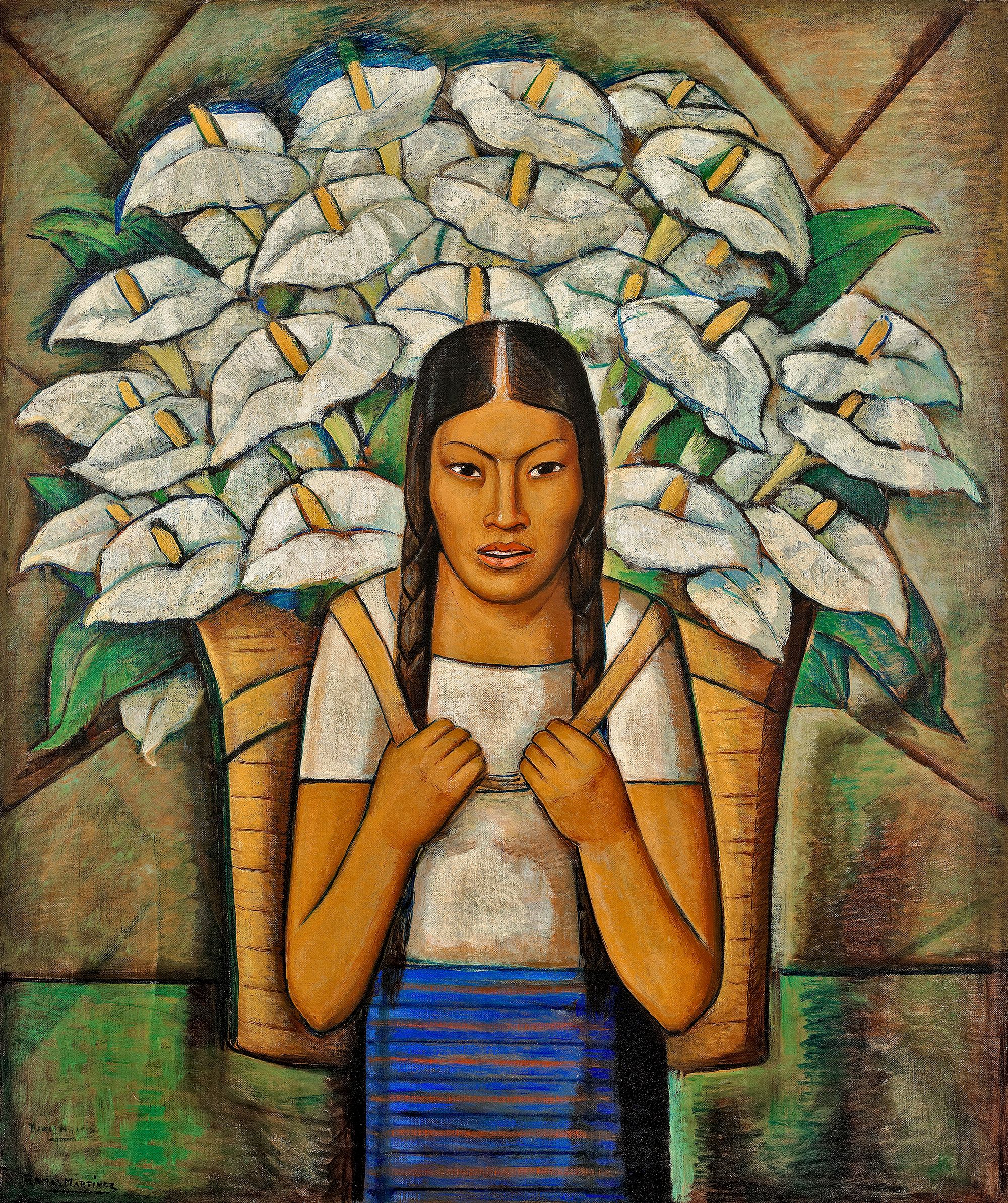The painting features an Asian woman facing forward, her long black hair parted down the center and styled into braids on either side. She is dressed in a white short-sleeved shirt paired with a blue and black striped skirt. Over her shoulders, she carries a large brown basket brimming with white calla lilies, which taper into green leaves and are accentuated by their yellow stamens. The oversized arrangement of flowers creates a dramatic arch above her head, dominating the composition. The backdrop is a wall rendered in shifting shades of beige and green, subtly enhancing the subject's presence.